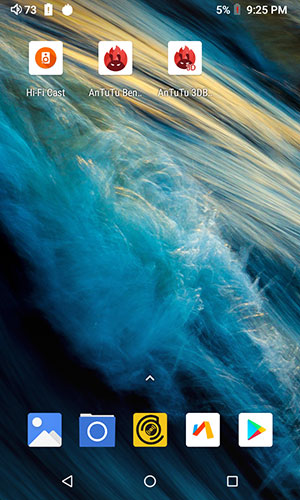This is a detailed screenshot of an Android device's home screen. The wallpaper features a mesmerizing long-exposure photograph of ocean waves, adding a serene and dynamic aesthetic to the display. 

At the top of the screen, there are three application icons, each characterized by white backgrounds and circular logos. The first icon is for HiFiCast, distinguished by an orange circle. Next to it, an app with "2-2-N" in its name is marked by a red circle. The third app, bearing "2-2-3-B-D" in its name, also features a red circle.

Further down, there are five additional icons grouped in a row. Among them are:
1. A Photos app, likely for managing and viewing images.
2. An app depicted by a picture icon.
3. A folder icon, possibly categorizing a group of apps.
4. A yellow icon that seems associated with music or records.
5. A unique logo with blue, red, and orange colors, which isn't immediately recognizable.

Prominently, the Google Play Store icon is also present, easily identifiable with its classic multicolored triangular design.

At the bottom of the screen, the familiar Android navigation UI is visible, providing access to essential controls for seamless device navigation.